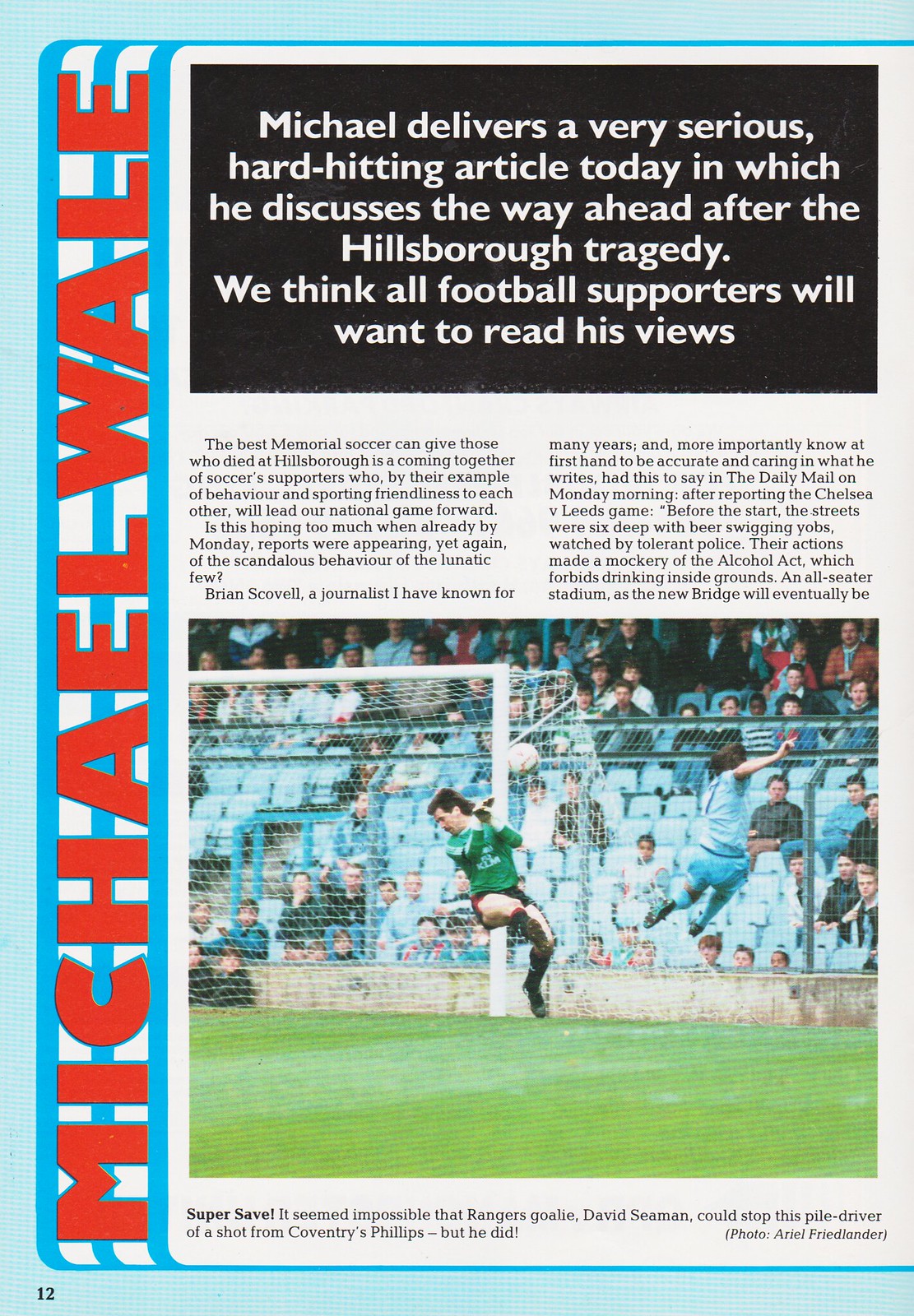This is a page from a game day program, specifically page 12, featuring a serious article by Michael Wale. The page is dominated by a black box at the top with white text, stating: "Michael delivers a very serious, hard-hitting article today in which he discusses the way ahead after the Hillsborough tragedy. We think all football supporters will want to read his views." The author's name, Michael Wale, runs vertically in red letters up the left side against a white and blue background. Below the black box are two columns of text, too small to read in detail. The lower half of the page is taken up by a dynamic photograph of Rangers goalie David Seaman in action. Wearing a green jersey and black shorts, Seaman is captured in the midst of making an impressive save, deflecting a powerful shot from Coventry's Phillips. The caption below the image reads: "Super save. It seemed impossible that Rangers goalie David Seaman could stop this pile driver of a shot from Coventry's Phillips, but he did." The page is bordered by a light blue margin, and the background includes spectators and a green playing field.